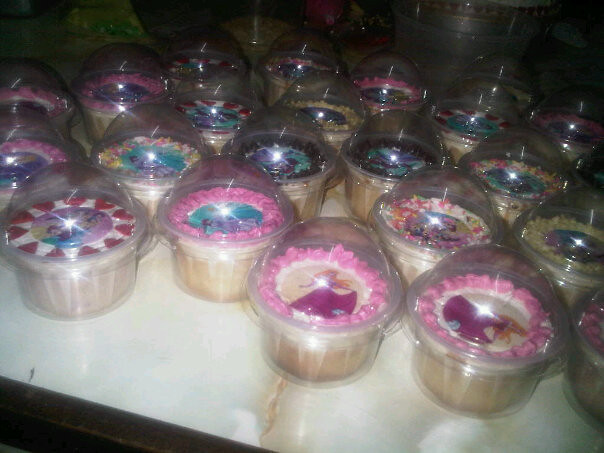This image captures an overhead, slightly side-angled view of a collection of intricately decorated cupcakes set on a white, marble-like table. The table edge, featuring brown trim with a black underside, is visible in the lower left corner. The background is slightly out of focus, showing hints of green and pink elements. 

Central to the photo is a large assortment of cupcakes, diagonally arranged from left to right, nearly covering the entire table surface. Each cupcake is nestled in a clear plastic dome container, with paper linings around the base to protect their delicate decorations during transportation. The cupcakes display a variety of designs, predominantly featuring shades of pink, purple, yellow, and white frosting, often adorned with sprinkles, fondant edges, or thematic figures. 

Many of the cupcakes are personalized with Disney princesses, including recognizable characters like Sleeping Beauty with her signature hot pink dress and orange hair, and Belle, surrounded by blue icing. Some appear to have red heart decorations and multi-colored sprinkles. The overall tone is festive, possibly prepared for a children’s party, indicated by the specific choice of princess-themed decorations.

The photo was likely taken at night, as indicated by the dark, flash-illuminated setting that highlights the colorful details of the cupcakes while casting darker shadows around the scene. This lighting suggests that the desserts were carefully prepared ahead of time, ready for the next day's celebration.